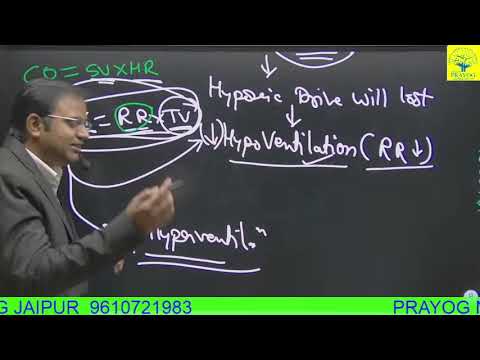The image depicts a Middle Eastern professor captured in profile, standing in front of a sleek, modern blackboard—likely a high-tech version allowing for marker use. He is wearing a brown suit jacket over a white collared shirt, has slicked-back black hair, and glasses. The professor is mid-sentence, holding what appears to be a marker in his right hand, suggesting he is in the midst of teaching. The blackboard behind him features two sections of writing: the far left corner has green text, while the majority of the board is filled with white writing, possibly mathematical or scientific notations. Along the bottom of the image, a neon green border displays blue numbers "96107 to 1983," and the names "Prayog" and "Jaipur" are visible, further hinting at the academic context. The image is framed with black borders at the top and bottom, suggesting it might be a still from an online video or YouTube channel.